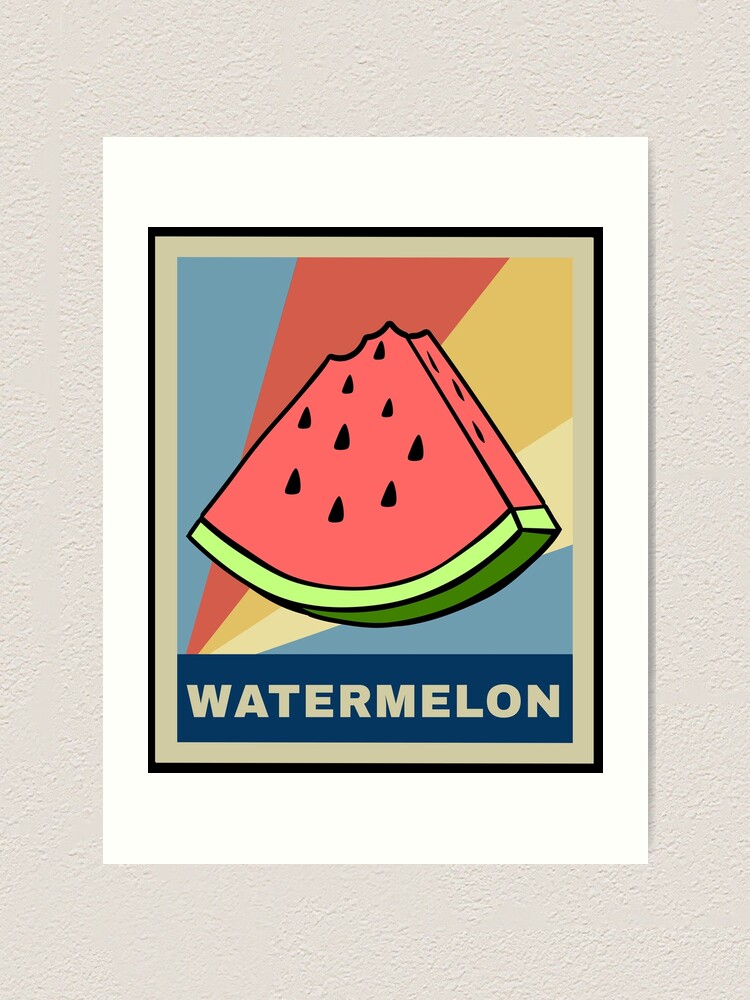This image features a framed piece of digital art styled after Andy Warhol's iconic 70s aesthetic. The focal point is a cartoonish, flat-colored slice of watermelon with a red interior, black seeds, and a green rind, complete with a bite taken out of the top. The word "Watermelon" is prominently displayed below the slice in a blue banner with beige lettering. A thin black frame encases the art, followed by a large beige matting. Behind the watermelon, a series of radiating rays of color—from red to gold to light gold—create a spotlight effect against a light blue background. The entire piece is set on a beige wall, giving the impression of how it might look when displayed.